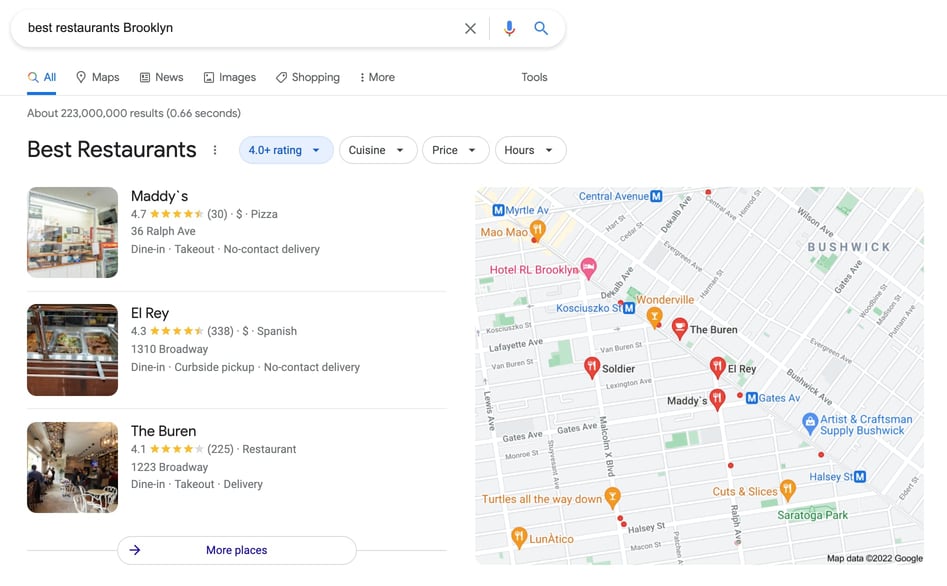This image is a screenshot of Google Maps displaying a search for the "best restaurants" in Bushwick, a neighborhood in New York City. On the right side of the screenshot is a map highlighting various food locations with red and orange markers, indicating the presence of restaurants in the area. On the left pane, a list of highly-rated restaurants is shown. 

Highlighted entries include:
1. **Maddie's** - Boasting a 4.7 rating from 30 reviews.
2. **El Rey** - Holding a 4.3 rating.
3. **The Burren** - With a significant 4.1 rating from 225 reviewers.

Each listed restaurant is accompanied by an image that provides a visual glimpse of the respective establishment. 

At the top of the screenshot, the search bar contains the query "best restaurants Brooklyn", which yielded 223 million results in just 0.66 seconds. At the very bottom of the image, there is a purple "more places" button, inviting users to explore additional options.

The map on the right clearly denotes the Bushwick area, offering a detailed geographical context for the restaurant search results.